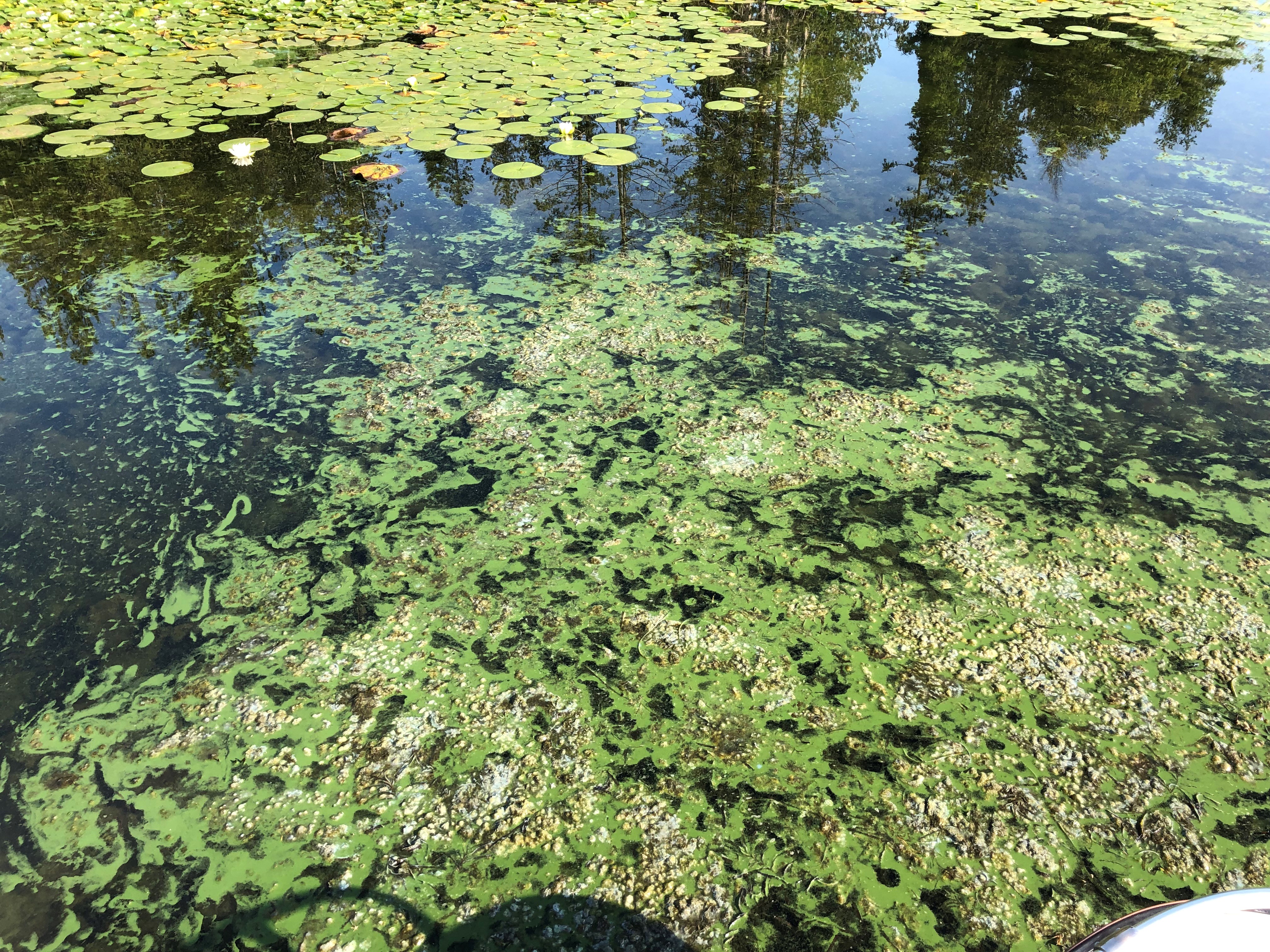The image is a close-up photograph of a pond with distinct layers of detail on its surface. In the background, the water is a dark gray color, predominantly covered by a mass of light green circular lily pads. Just below these lily pads, you can observe the reflection of tall pine trees. Moving closer to the foreground, a slimy layer of light green algae or pond scum covers a major portion of the water's surface, interspersed with off-white, puffy bits that could be frog eggs or tadpoles. In between the lily pads and the algae, there are clear sections of the pond where the surface water reflects the surrounding trees. At the very front, some floral elements or fragmented leaves float on the water, while a small shadow at the bottom might suggest the presence of the photographer. This overall intricate scene mirrors the serene and slightly eerie ecology of a pond, emphasizing its layered and reflective qualities.